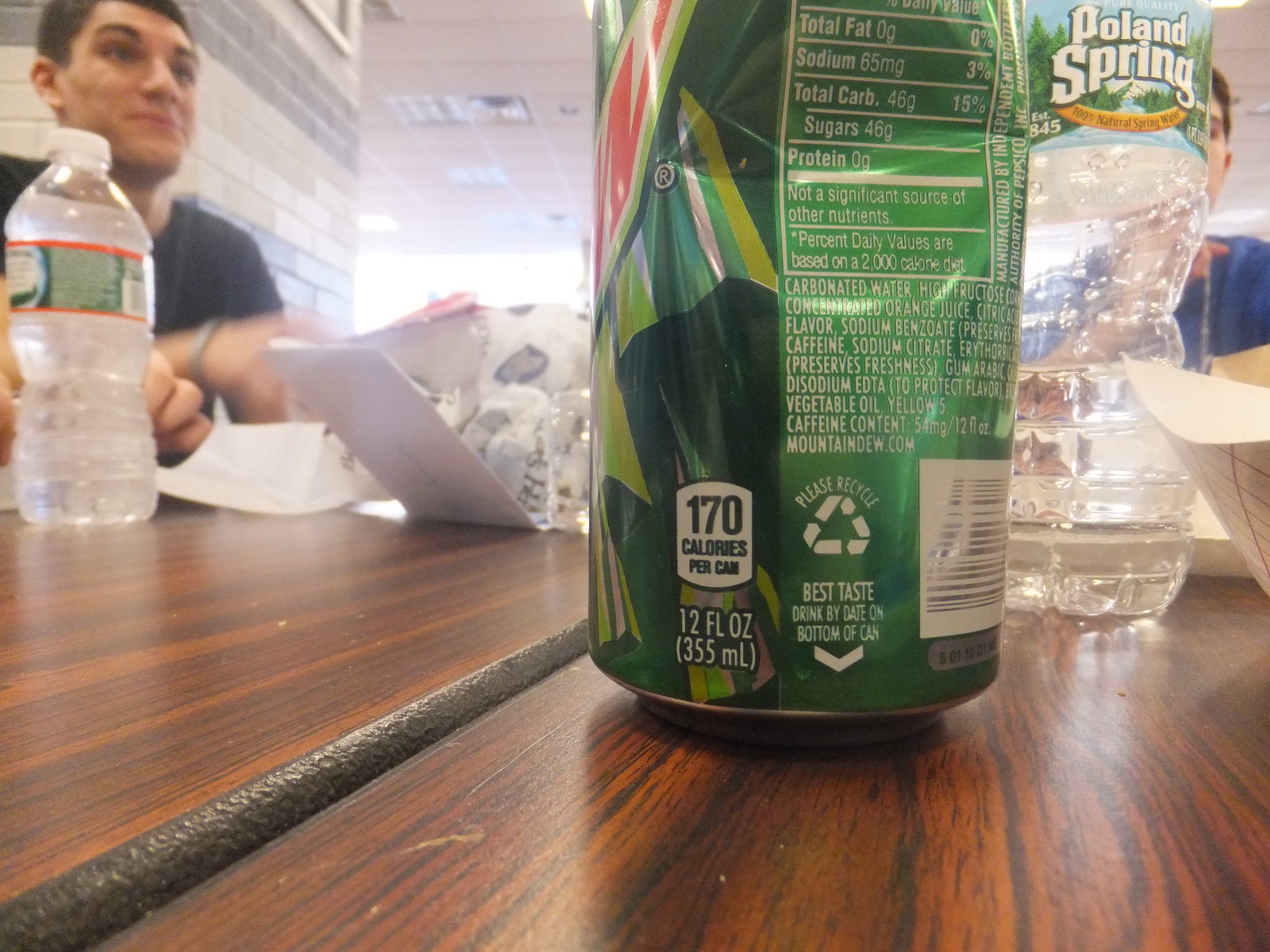This vibrant color photograph provides an intimate, close-up view of a faux wood table, with dark and medium brown tones. The camera angle is set as if it were placed on the table, creating a dynamic perspective. Dominating the foreground is a slightly dented can of Mountain Dew, showcasing its dark green, medium green, yellow, and silver colors. The back of the can is visible, revealing nutritional information, including the 170-calorie count, and the white recycling symbol.

Behind the can, a clear Poland Spring water bottle with a white cap and green and red label is discernible. Another empty Poland Spring water bottle is positioned towards the right side. To the far side of the table, there is a partially visible man with short dark hair, wearing a black short-sleeved t-shirt. In front of him is another clear water bottle with a green label. In the background, gray and white striped tile walls and a drop ceiling with lights and fans add context and depth to the scene.